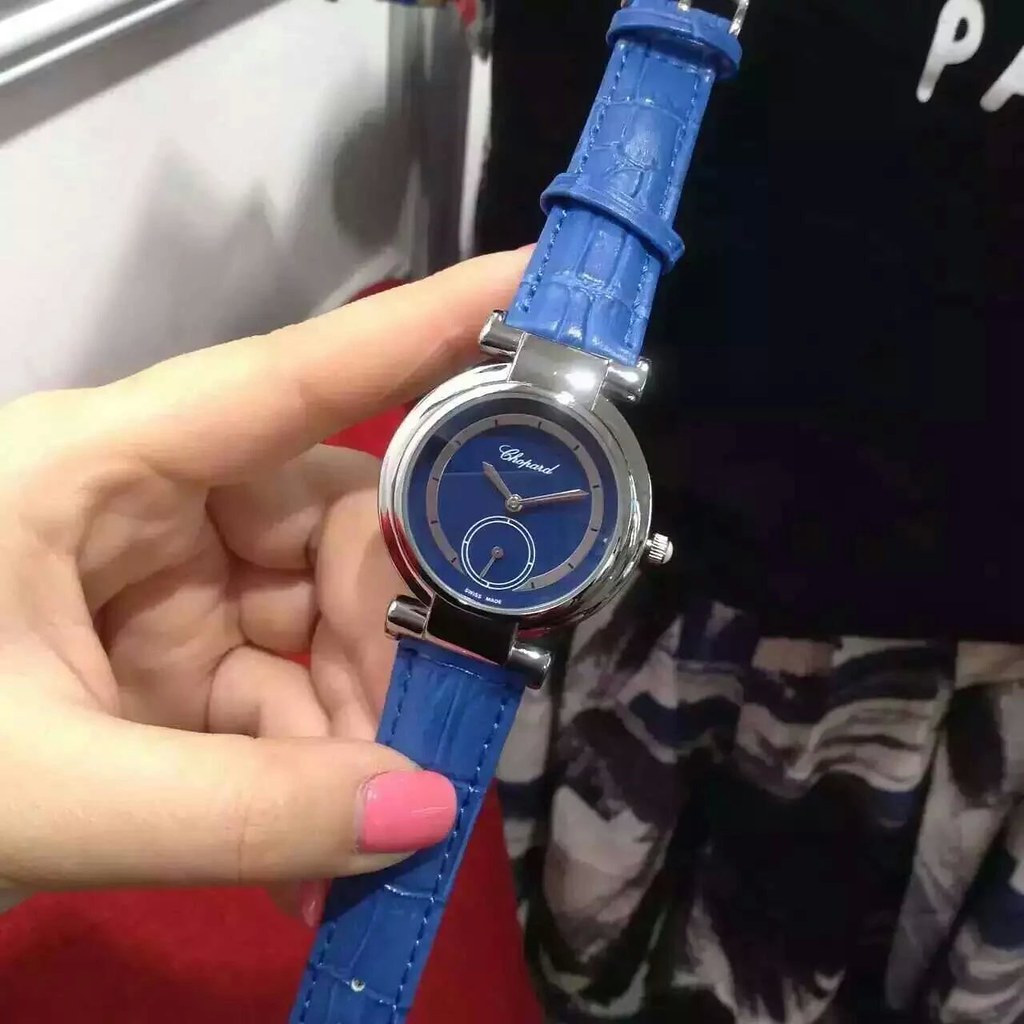In this close-up shot, a woman's hand, showcasing long slender fingers with nails painted pink, delicately holds a wristwatch. The watch's silver case gleams under a bright overhead light, enhancing the elegant design. The watch face displays a rich dark blue color, adorned with slender silver hands and small notches replacing traditional numbers. At the bottom of the face, a subsidiary dial features an additional needle for the seconds. Encircling the blue face is a silver border, adding a refined touch. The brand name "Clepard" is subtly inscribed in white. The wristband, made of bright blue leather with an alligator texture, is fully visible as the watch lies flat in her hand. In the blurred background, the silhouette of an individual dressed in a black skirt and top can be discerned, adding a contrast that further highlights the watch.